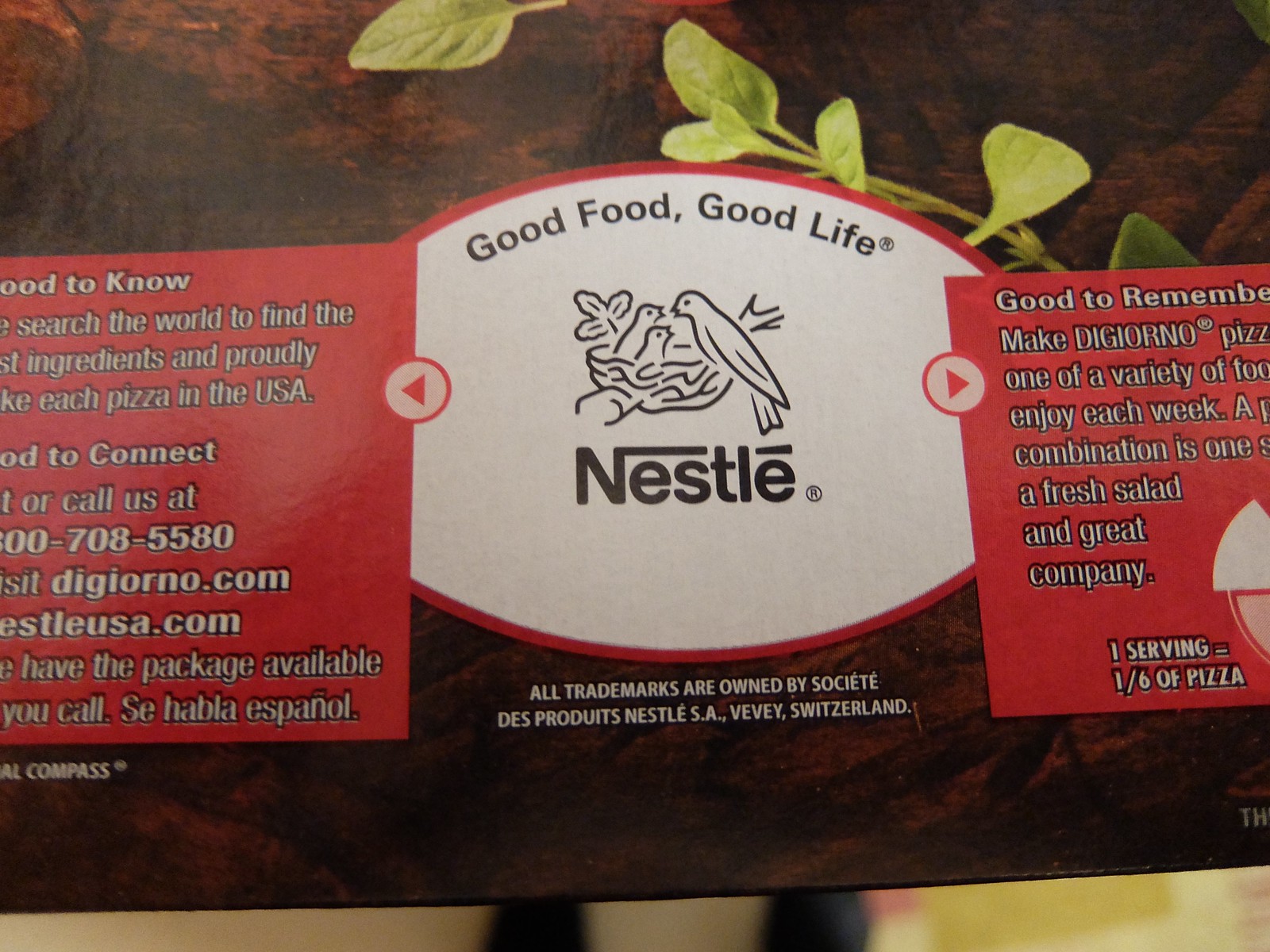A close-up photograph of the back of a DiGiorno pizza box made by Nestlé. Dominating the center of the image is the Nestlé logo, featuring the company name in white text and a few bird illustrations above it. Below the logo, the slogan "Good Food, Good Life" is prominently displayed. On the right side of the box, there's a red section with white text encouraging customers to "Make DiGiorno Pizza," accompanied by nutritional information that states one serving is one-sixth of the pizza. The left side features another red box also containing various texts, including customer service details and trademarks associated with Switzerland. The overall design is clean, with the white Nestlé logo standing out against the red background, surrounded by information relating to pizza servings and company contact information.